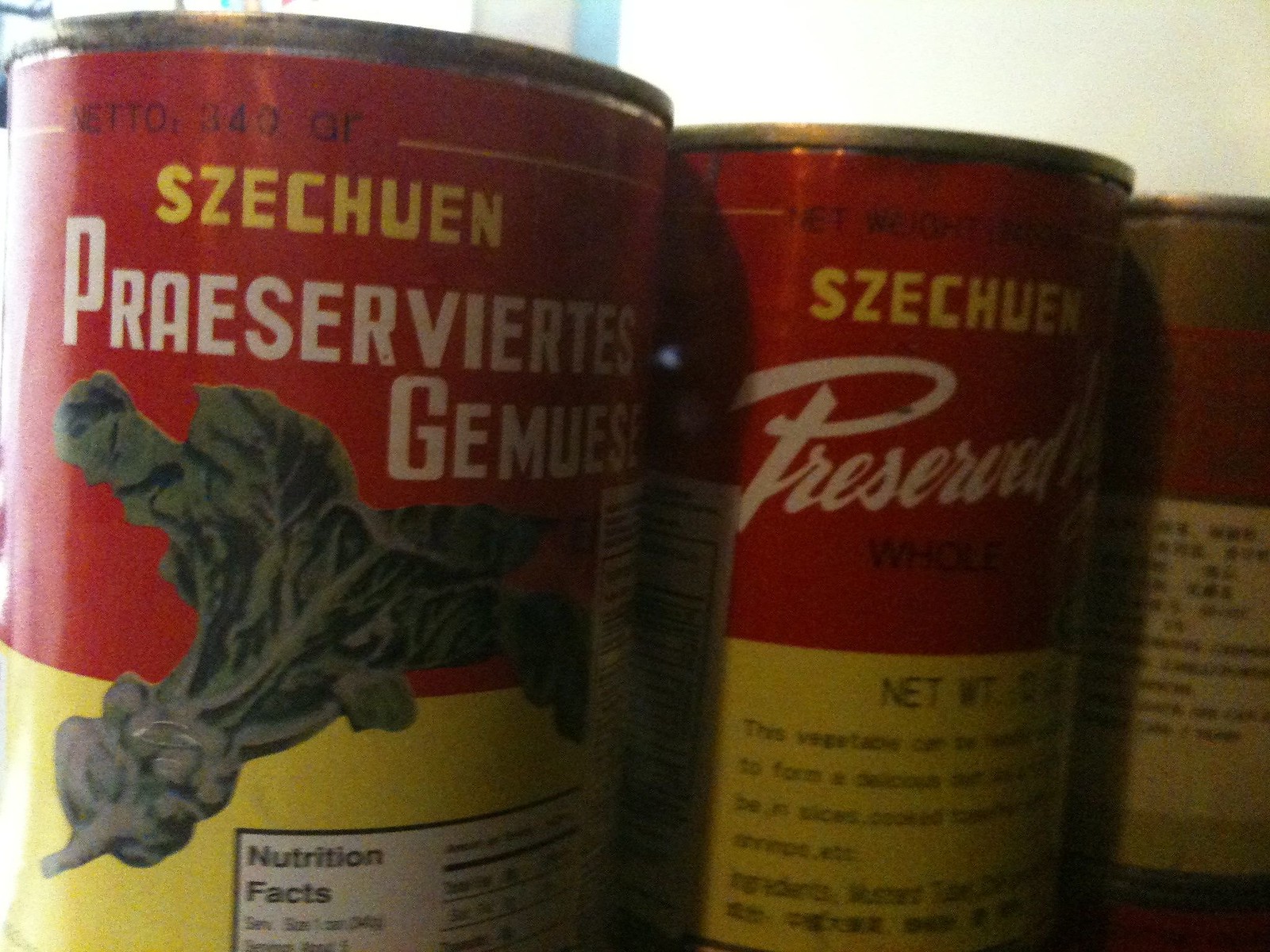This photo showcases three old-fashioned cans from Sichuan Preserve, labeled as "Jammus." The labels feature a vintage design with a solid red and yellow background, complemented by an antique-style illustration of a green leafy vegetable. The first can's front prominently displays the nutrition facts, while the second can provides details about the net weight and ingredients. The third can includes some Chinese characters. The image is slightly blurry, adding to the overall aged appearance of the cans.